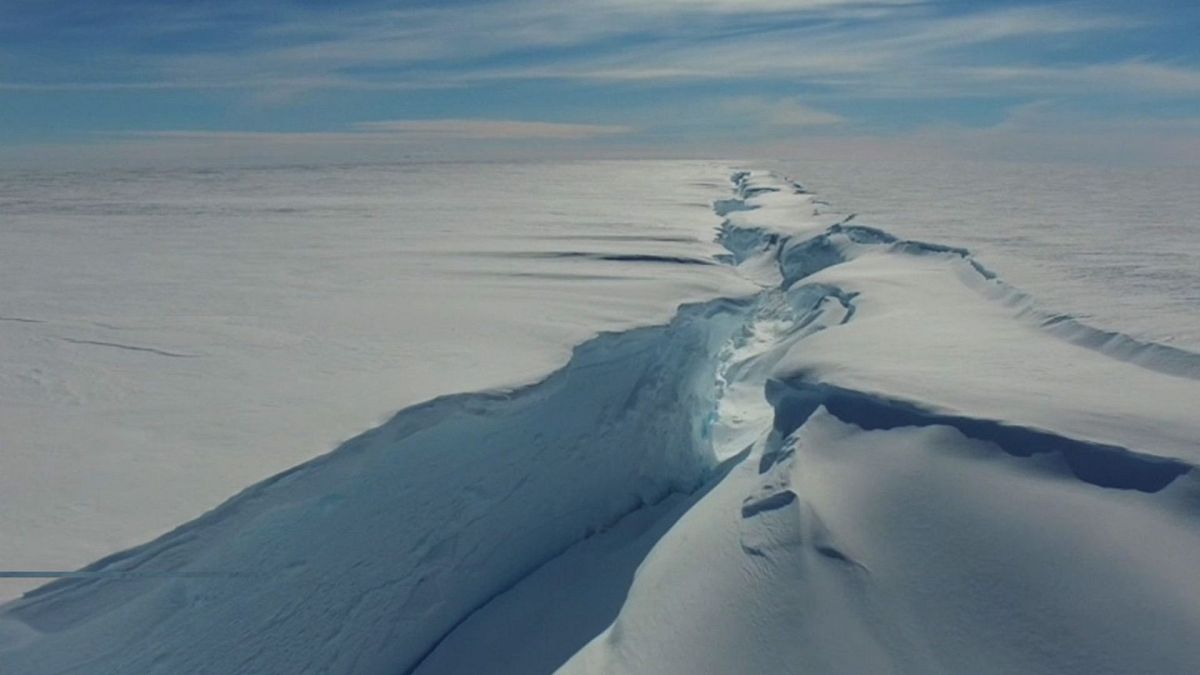This image showcases an expansive, icy landscape dominated by a massive mound of deep snow, seemingly endless and imposing. The snow cover is incredibly thick, almost bluish in hue, indicating it has accumulated over a long period. A significant separation or crack bisects the snow, creating a steep, wall-like division, possibly suggesting a glacier or ice field breaking apart. Above this frigid scene, the sky stretches across the top section of the image, a medium blue adorned with wispy white clouds in a horizontal formation. The overall composition is horizontally-oriented, embodying the vastness of this cold, snowy terrain with additional stretches of icy land extending to the left and right. The entire scene evokes the enduring and harsh beauty of a frozen landscape.